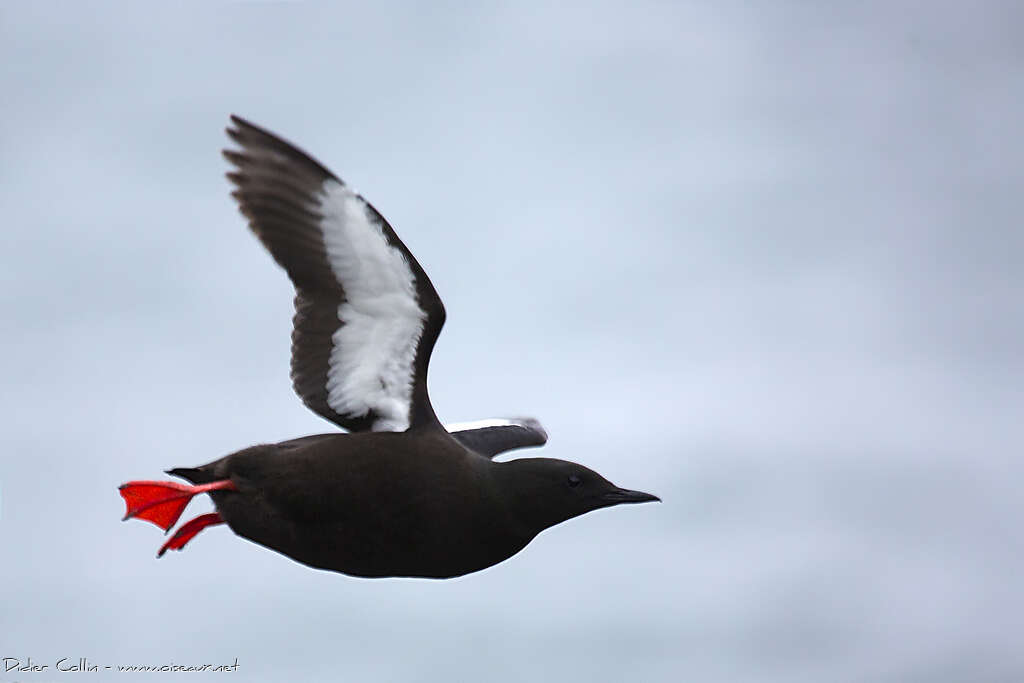The image features a striking black guillemot in mid-flight against a vast, grayish-blue sky that dominates the background. The bird's large wings are spread wide, revealing a mix of white and black feathers. Its right wing is more prominently displayed, with white feathers visible underneath, while the left wing shows only a glimpse of its white-tipped feathers. The guillemot’s sharp, dark beak points to the right, and its bright red, webbed feet extend to the left. The bird's body is predominantly black with a slight hint of brown. At the bottom right corner of the image, there's a small, hard-to-read text that likely includes a copyright symbol, the artist's name, and possibly a website address. The sky, filled with clouds, provides a blurred, muted backdrop that makes the bird’s detailed features stand out prominently.